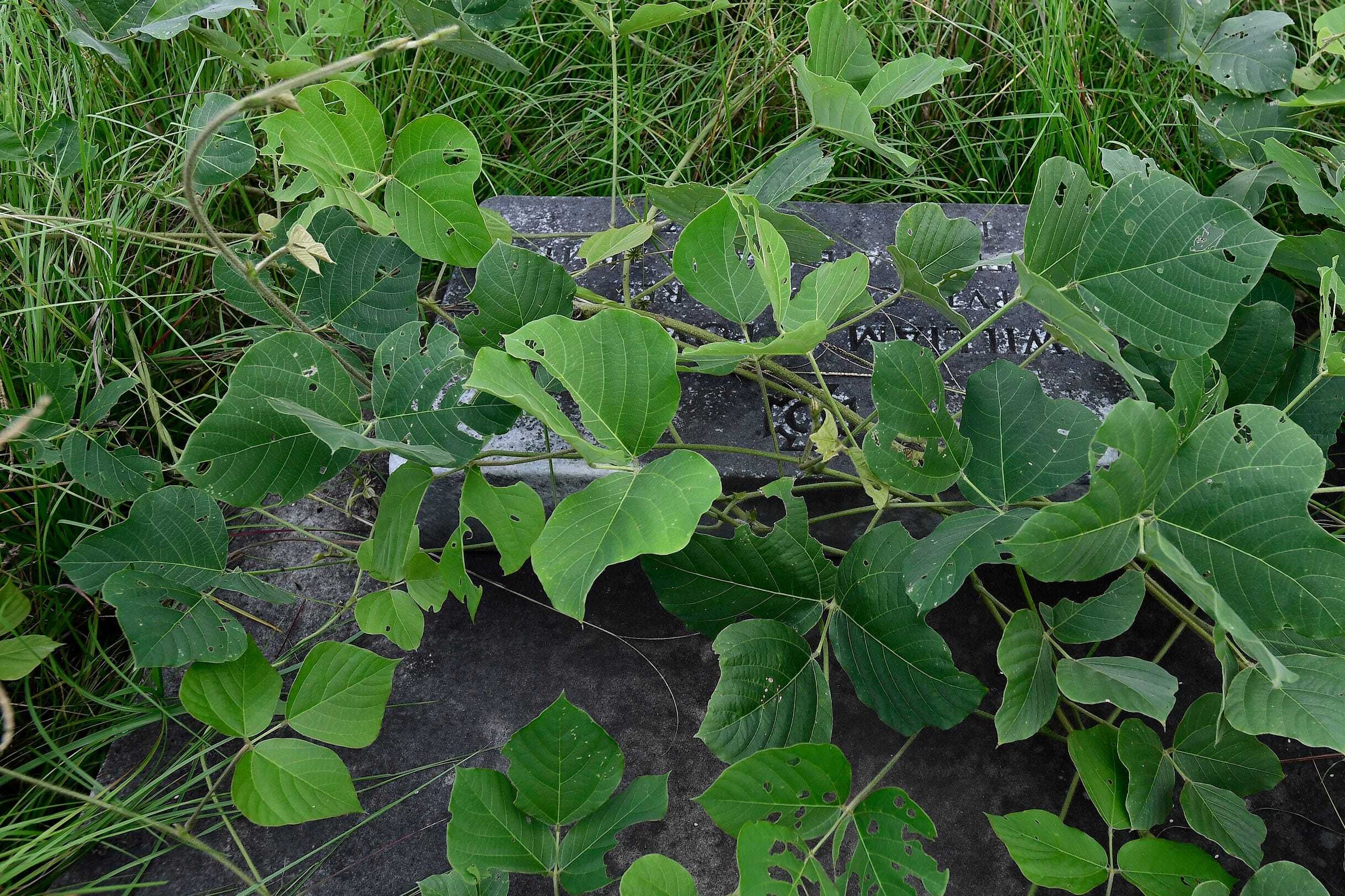The image depicts an outdoor scene featuring a weathered gravestone, partially veiled by a dense layer of tall, unkempt grass, leaves, and overgrown vines. The photograph, taken from a top-down perspective, offers a rectangular frame where the gravestone is centrally focused. Although the stone appears predominantly gray through the passage of time, hints of its original white hue are still visible. The engraved text on the stone is largely obscured by the thick vegetation, with only a small cross at the bottom center faintly discernible. A mix of green from the grass, browning stalks, and the dark, earthy tones of the dirt around it create a somber and abandoned atmosphere. The image emphasizes the neglect and natural reclaiming of what might be a historically or personally significant site.